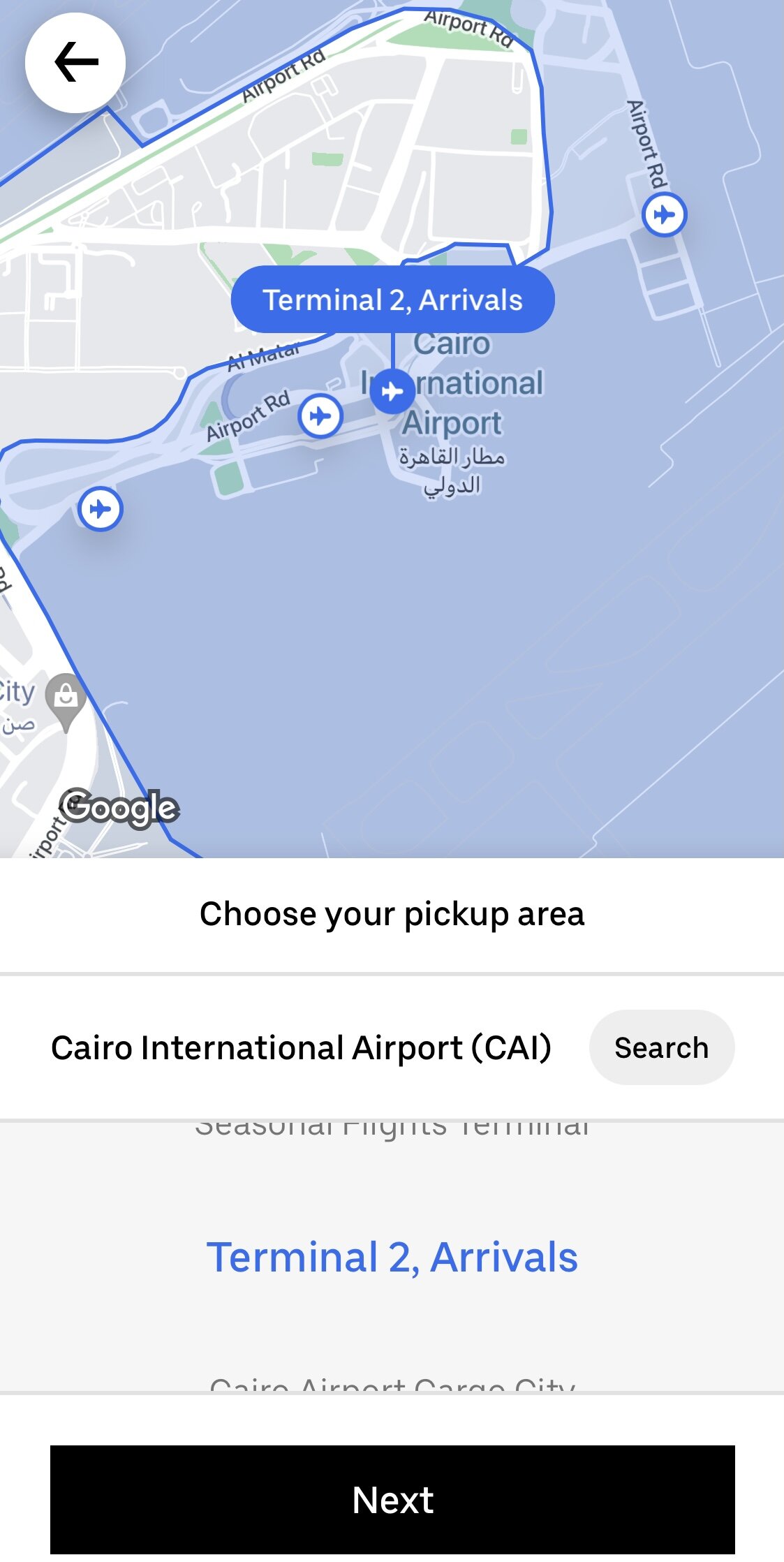A screenshot from an airport navigation app, likely depicting Google Maps, centers on Cairo International Airport (CAI). The map displays major routes such as Airport Road and highlights significant areas within the airport. One prominent feature is Terminal 2 Arrivals, marked with a blue capsule shape and a plane icon. The map's overlay provides a top-down view of the airport, with what appears to possibly be bodies of water indicated by blue areas, although this is not entirely clear.

Beneath the map, there is a user prompt: "Choose your pickup area." This area is demarcated with thin gray lines and includes a drop-down menu and a search button adjacent to "Cairo International Airport (CAI)." Below this are selectable options, with "Terminal 2 Arrivals" highlighted in blue text. The scrolling list also hints at other areas such as the "seasonal flights terminal," though it is partially obscured.

At the bottom of the screen, the text is partially cut off but references locations like "Cairo Airport" and possibly "Cargo City." Dominating the lower portion is a large black rectangle featuring the word "Next" in white, indicating a navigation button. The familiar Google logo can be seen in the bottom left corner of the map.